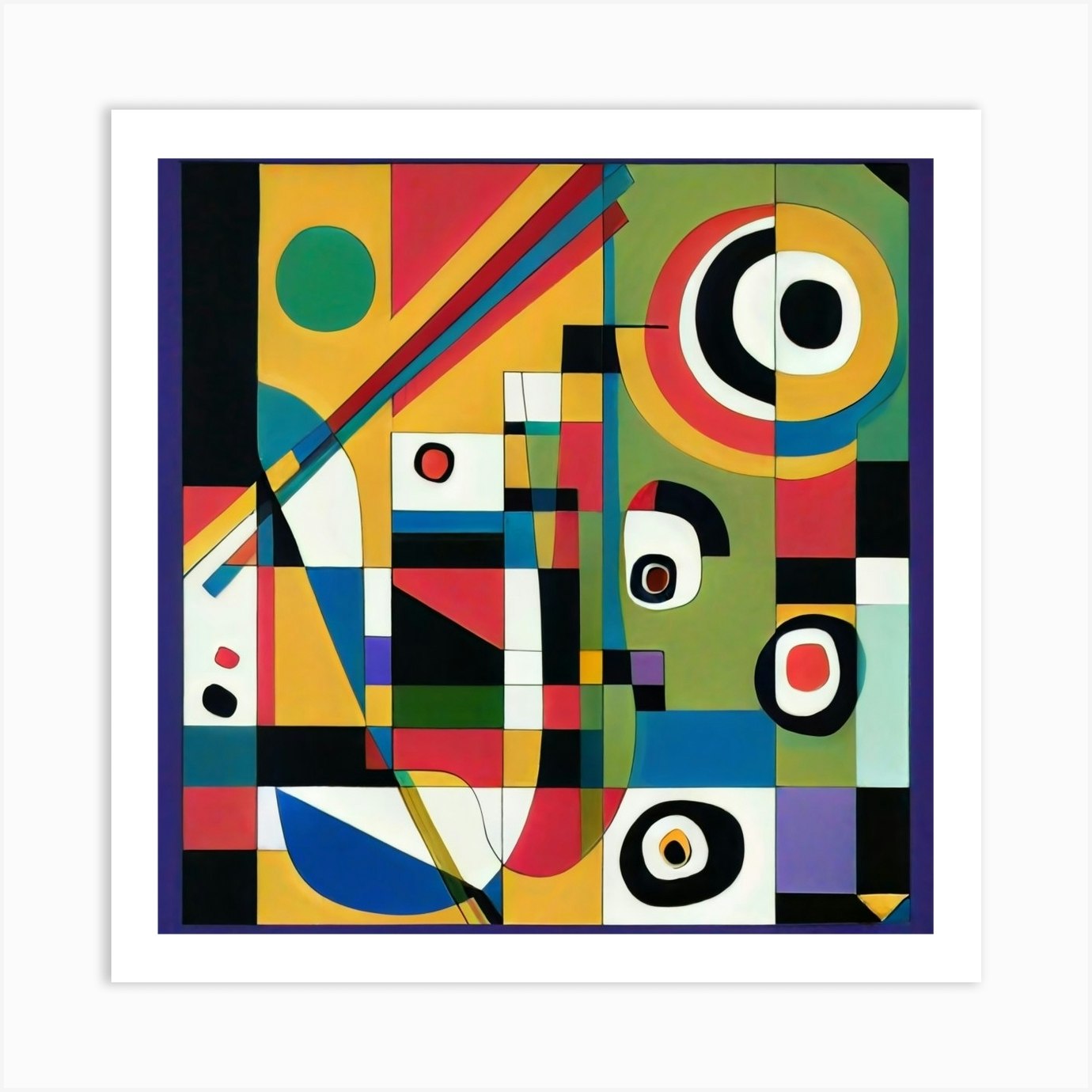The image is a square-shaped abstract painting framed by a white border. Inside, a diverse array of geometric shapes such as rectangles, squares, triangles, circles, and half-circles dominate the composition. These shapes are arranged in a seemingly random pattern and feature a wide range of colors including black, white, yellow, green, blue, purple, pink, and some red. The transitions between the shapes are marked by different colors, creating a patchwork effect. The painting also has a distinctive purple border on all sides except for the top. The shapes and colors are distributed in columns but do not form any recognizable object, adding to its abstract nature. Some elements resemble eyes and chopsticks, adding a sense of whimsical disorder to the piece. The overall color palette is rich and dark, making the vibrant interplay of colors stand out against the off-white background.